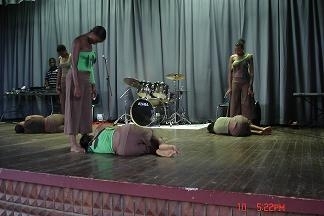This photograph captures a stage scene with intricate details and multiple figures engaged in a performance. Dominating the stage are three women standing, each looking down with their heads bowed towards another three women who are lying prone on the ground, legs folded in fetal positions. All six of these individuals are barefoot and dressed in gray pants and green tops, creating a visually cohesive group that could be portraying an Egyptian theme. 

At the backdrop of the stage, a gray curtain hangs down, partially covering a drum set placed on a white platform. To the far left, a dark-skinned man stands behind a table or desk, although his exact role remains unclear due to distance; he might be a DJ or part of the crew. The stage itself is wooden and dark, with a carved bottom edge accentuated by a red band running along the top. Some time code reading "522 PM" is visible at the bottom of the photograph.